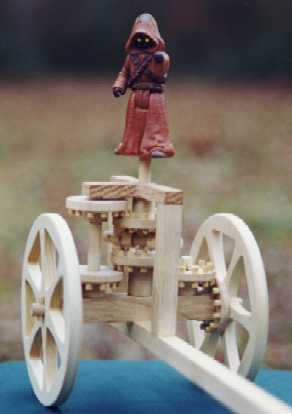The image depicts a detailed miniature wooden wagon with two wheels on either side and a long pole extending diagonally to the bottom right corner. This intricately crafted wagon, resting on a blue table, features gears, suggesting it's part of a functional or mechanical hobby piece. Standing on the wagon is a small figurine, dressed in a red hooded robe that covers its entire body, and black gloves. The figure's face is entirely black except for two yellow eyes, and it has two black straps crisscrossing on its chest. The background of the image is blurry, but hints of green and brown suggest the presence of trees or foliage, adding a natural setting to the scene.